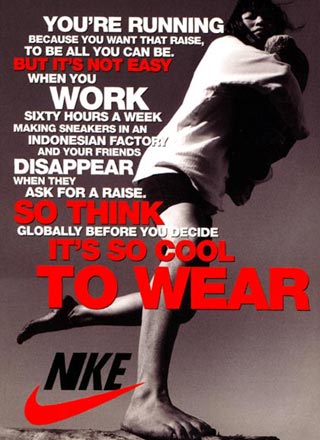The image is a poignant, grayscale advertisement that criticizes Nike's labor practices. It features an African American woman standing on a rock, barefoot, elegantly balancing on one leg with the other leg lifted and toes pointed back. Her arms are crossed in front of her, and she's gazing forward. She’s dressed in an oversized, light-colored long-sleeve shirt and dark shorts that reach halfway down her thighs.

Text in bold white and red capitals overlays the image, creating a stark contrast against the gray background. The top of the image reads, "You're running because you want that raise to be all you can be." Below, red text states, "But it's not that easy," followed by white text detailing the harsh realities: "when you work 60 hours a week making sneakers in an Indonesian factory and your friends disappear when they ask for a raise." It concludes with a powerful admonition in alternating red and white text: "So think globally before you decide it's cool to wear." At the bottom, the Nike logo and its red swoosh serve as a chilling reminder of the brand's alleged ethical shortcomings.